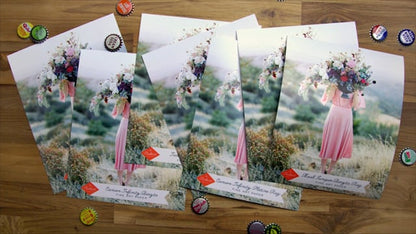This detailed photograph showcases multiple prints of a single image laid out on a light brown wooden table, where the wood grain is distinctly visible. The images, totaling around six or seven, are slightly overlapping each other. Each print features a woman in a pink dress standing on a grassy hillside. Her face is obscured by a bouquet of vibrant flowers in a planter, featuring red, purple, pink, and white blooms. Below the image, there is a white banner with black cursive text, although it is too blurry to decipher.

Surrounding the photographs on the tabletop are various bottle caps, adding colorful details to the composition. Notably, there is a Mike's Hard Lemonade cap at the bottom, a Pepsi cap towards the upper right, and other caps in a range of colors including red, green, yellow, silver, and black, each with distinct markings that are hard to read. The arrangement of bottle caps—red with white letters, green with dark green letters, yellow with red letters, and others—complements the scattered layout of the photos, creating a vibrant and eclectic scene.